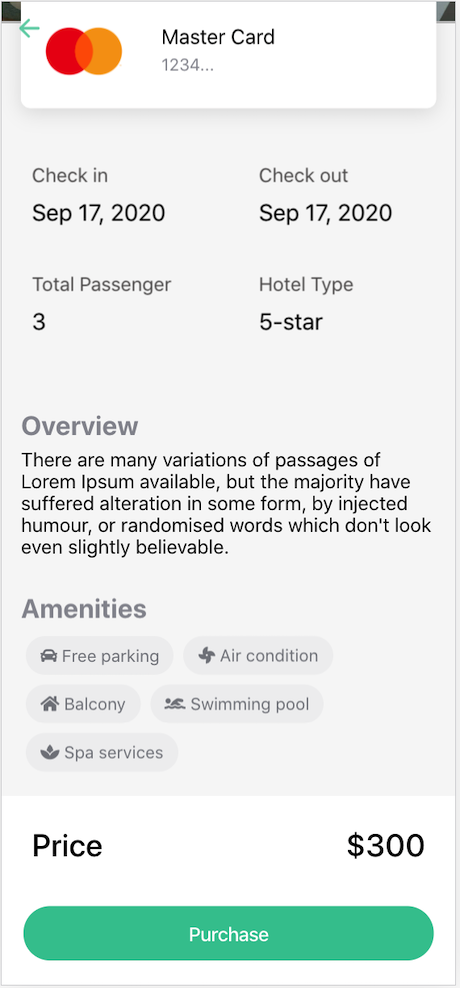This image is a screenshot from a smartphone displaying a hotel booking template. At the top of the screen, there is the MasterCard logo, featuring a red oval overlapping a yellow oval, with the text "MasterCard" centered beneath it. Below the logo, the placeholder credit card number "1234" is shown.

The background of the page is light gray. The check-in date is listed as "September 17, 2020," and the check-out date is the same. The next section details the total number of passengers, which is three, and specifies a five-star hotel type.

This appears to be a template, not an actual payment page, as indicated by the section titled "Overview." This section contains placeholder text that begins with "There are many variations of passages of," followed by additional dummy text meant to simulate final content.

Further down, the "Amenities" section lists features of the hotel: free parking, air conditioners, balconies, a swimming pool, and spa services. At the bottom of the screen, the price is displayed as "$300." A purchase button, in aquamarine green with rounded edges and white text, is positioned at the bottom, labeled "Purchase."